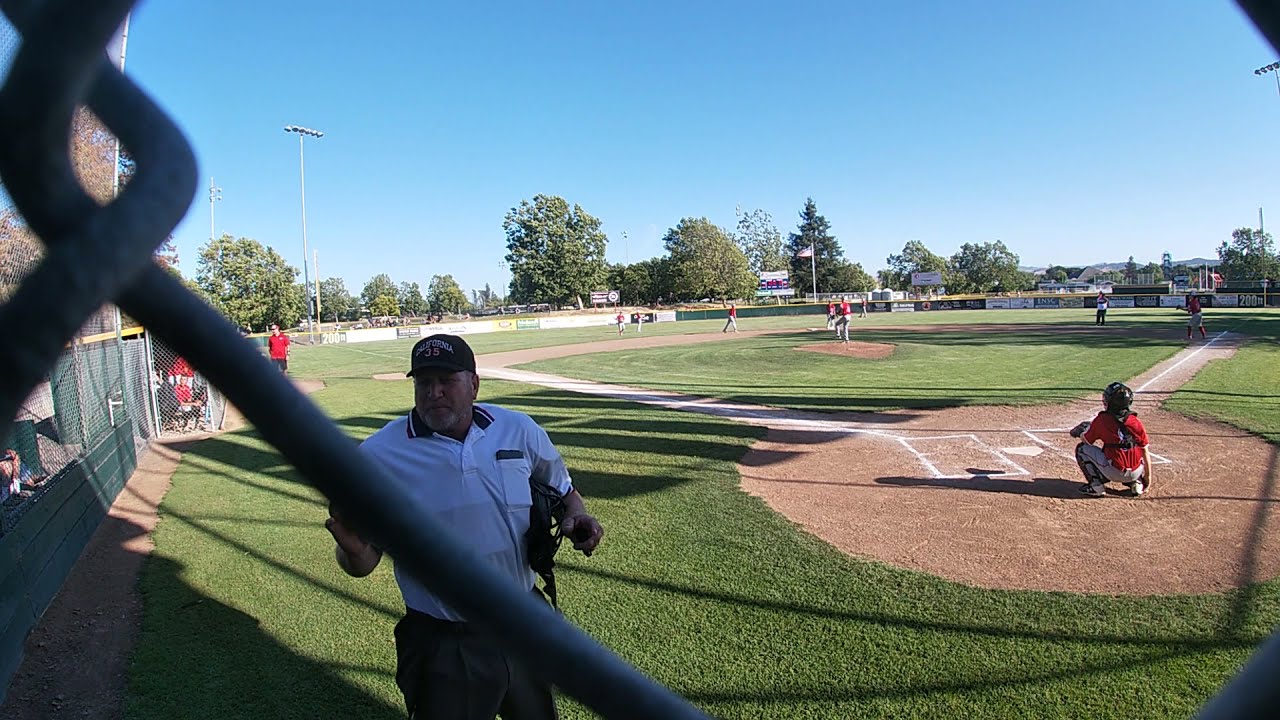This horizontally aligned, rectangular photograph captures a vibrant outdoor baseball field on a clear, sunny day. The top of the image reveals a striking blue sky free of clouds. Along the horizon, a variety of trees with lush green leaves, including tall and round types, as well as some with a Christmas tree shape, create a scenic backdrop. The field is enclosed by a chain-link fence, noticeably visible as it descends diagonally from the upper left to the lower middle of the image.

In the foreground, we're looking through this fence at an umpire standing on the near side, almost facing us. He is dressed in a white polo shirt with a black collar, a black baseball cap with indiscernible writing, and gray pants. He holds a mask in his hand, suggesting he's preparing for the game. Nearby, on the right side, a catcher in a red jersey and white pants is positioned, facing the field. His attention is directed toward the pitcher, whose leg is raised as if in mid-throw, also sporting a red jersey and white pants.

The green grass contrasts sharply with the brown soil and white chalk outlining the baseball diamond. Further back, you can discern a few players scattered in the outfield. Tall lights and even an American flag on a pole can be seen in the distance, though the lights remain off. The presence of only one team suggests this could be a practice session. The composition beautifully captures the essence of a sunny day at the baseball field, framed by the natural and structural elements that define the scene.